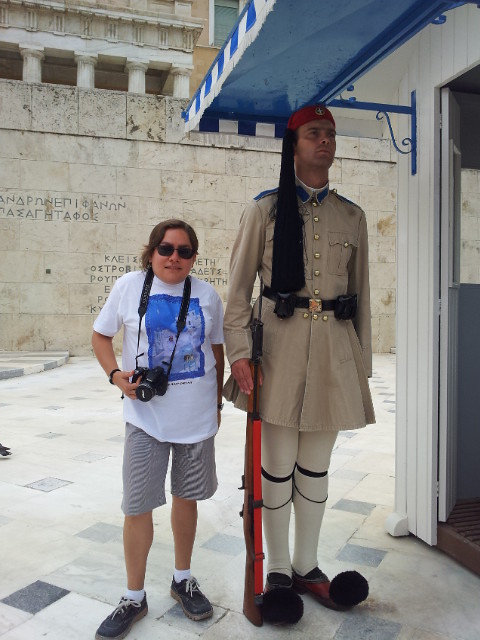In this photograph, a tourist and a ceremonial guard stand side by side against the backdrop of an ancient Greek building adorned with columns and a stone wall engraved with Greek text. The tourist, on the left, poses confidently in a white graphic t-shirt with a blue design, gray shorts, and black sneakers featuring white laces and brown bottoms. A black camera, hanging from a strap around their neck, rests in front of them, and they wear a wristwatch on their right wrist and black rimmed sunglasses shielding their eyes. 

To the right, a tall guard in an elaborate ceremonial uniform stands at attention. The guard's attire includes a tan calf-length tunic with blue lapels and collar, adorned with brass buttons and chest pockets. A leather belt with small cases wraps around the waist. The uniform is completed with white stockings and black shoes accented by black pom-poms on the toes. A red hat with a black tassel and a long banner adds a vivid splash of color, while a rifle with a red strap rests against the guard's shoulder, its butt on the ground. The scene is a striking juxtaposition of modern casual attire and historic ceremonial regalia.